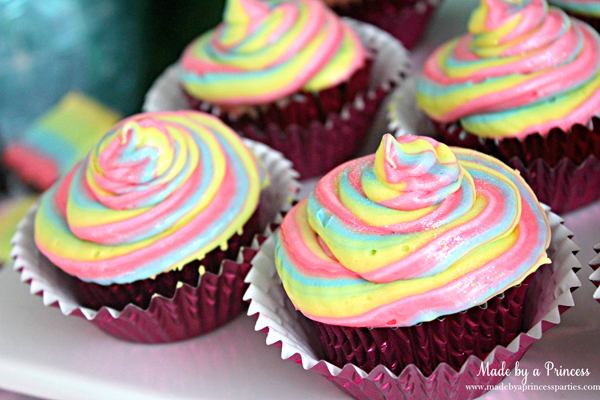This vibrant photograph features an assortment of stunning cupcakes, elegantly showcased on a glossy white tabletop. Each of the four visible cupcakes is nestled in a rippled, shiny pink foil cupcake holder, accentuating the luxurious presentation. The cupcakes themselves appear to be chocolate, beautifully adorned with a luscious swirl of icing in a mesmerizing blend of pink, yellow, and blue, creating an enticing marbled effect that even hints at shades of green where colors mix. The bottom right-hand corner of the image bears the branding "Made by a Princess," accompanied by the website www.madebyaprincessparties.com, suggesting a professional, whimsical touch suggestive of a delightful confectionery business. The background remains softly out of focus, allowing the eye-catching details of the cupcakes to stand out vividly.